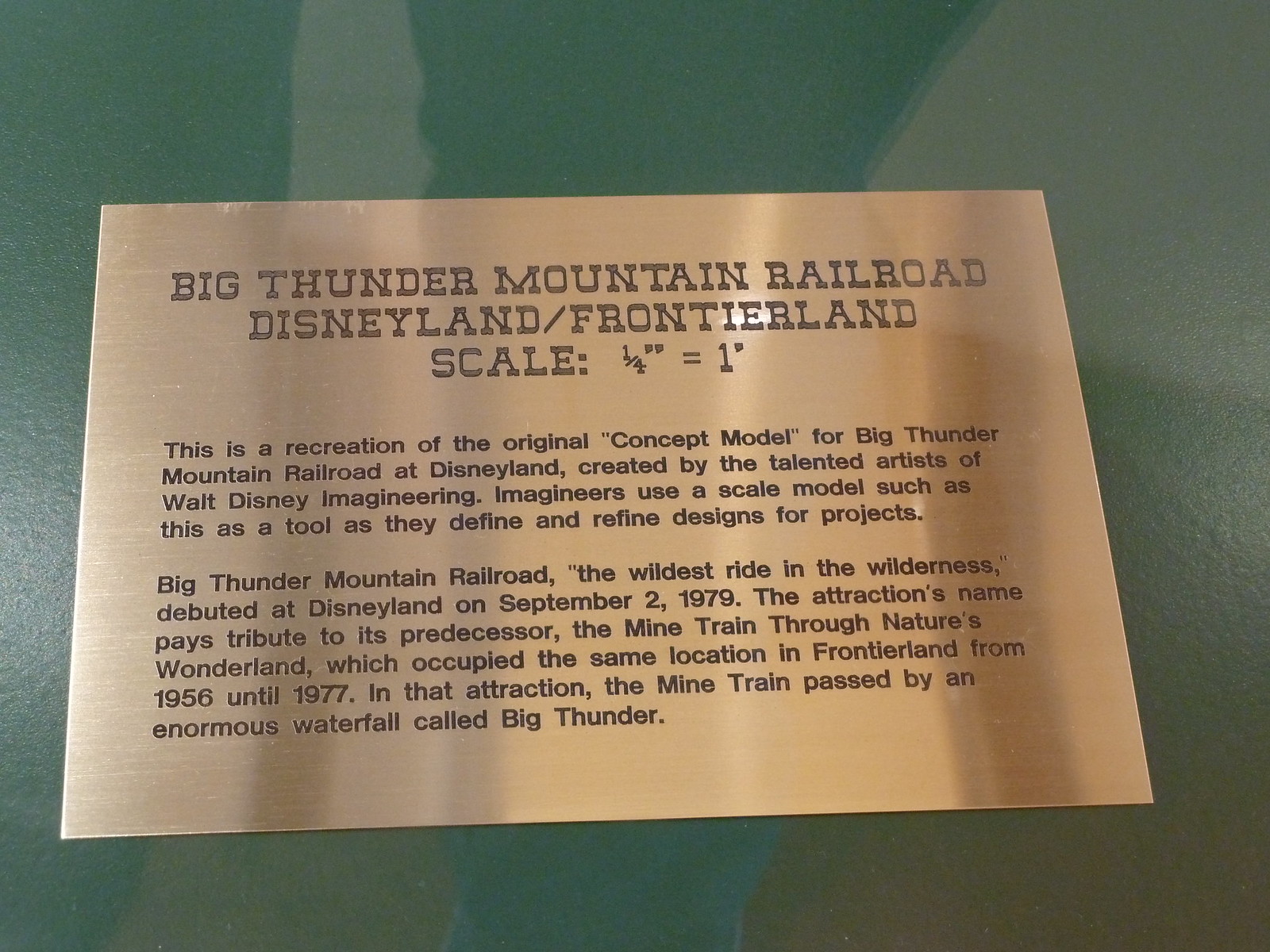This image showcases an informational plaque that serves as a part of an exhibit at Disneyland. The plaque, which appears to be made of stainless steel with engraved text that shimmers, is titled "Big Thunder Mountain Railroad, Disneyland / Frontierland" in dark brown letters against a lighter brown background. The scale mentioned on the plaque is "1/4 inch equals 1 foot." The text beneath the title reads: "This is a recreation of the original concept model for Big Thunder Mountain Railroad at Disneyland, created by the talented artists of Walt Disney Imagineering. Imagineers use a scale model such as this as a tool as they define and refine designs for projects." The plaque also provides historical context, stating, "Big Thunder Mountain Railroad, the wildest ride in the wilderness, debuted at Disneyland on September 2nd, 1979. The attraction's name pays tribute to its predecessor, the Mine Train Through Nature's Wonderland, which occupied the same location in Frontierland from 1956 until 1977. In that attraction, the mine train passed by an enormous waterfall called Big Thunder." The plaque is set against a glass background and identifies the scale model associated with the Big Thunder Mountain Railroad exhibit.